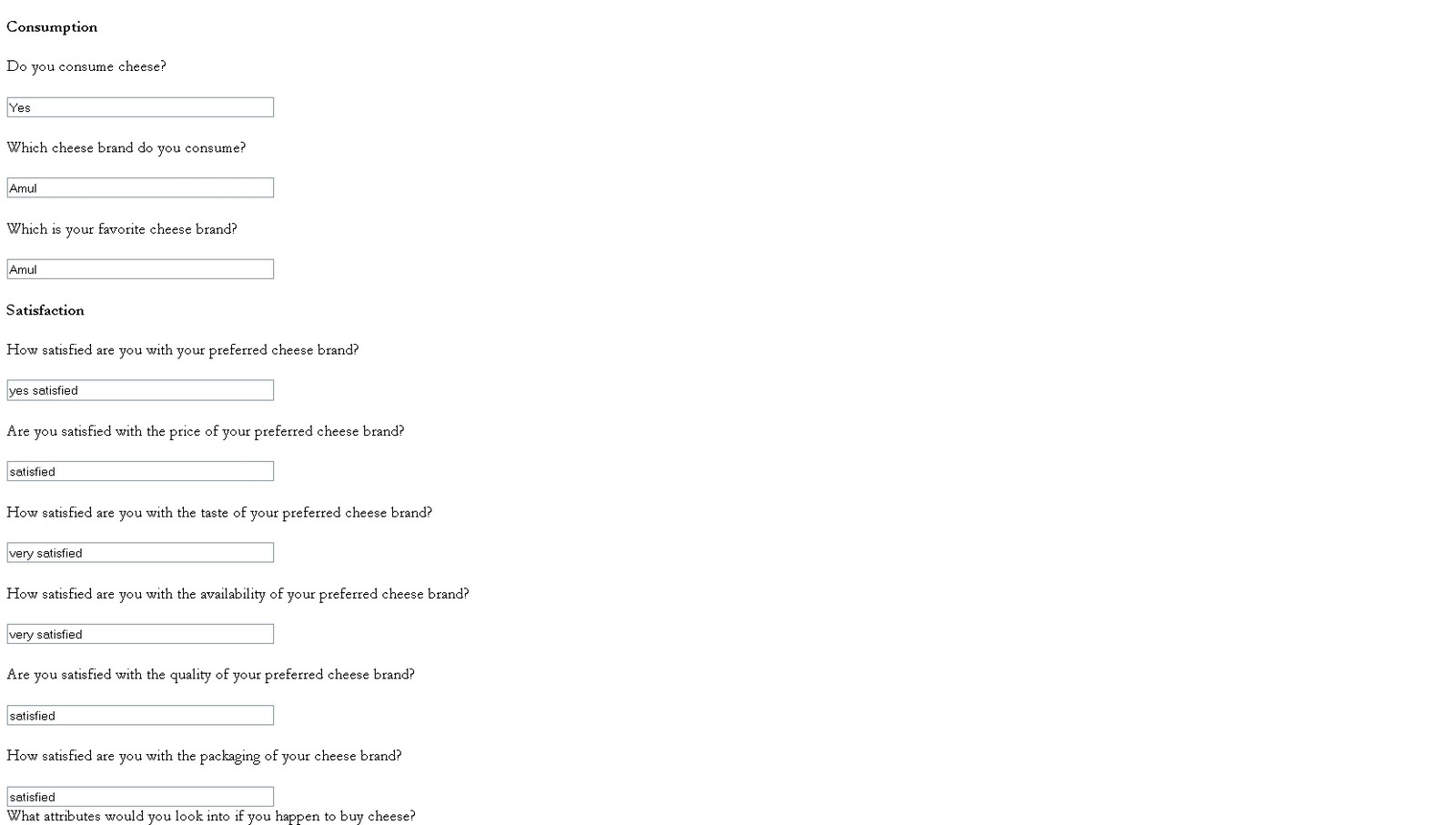The image depicts a survey form focused on cheese consumption, presented in a straightforward table format. The header, in bold print, reads "Consumption". The survey consists of various questions designed to gather detailed information about the respondent's cheese preferences and satisfaction levels.

- **Question 1:** "Do you consume cheese?" 
  - **Response:** "Yes"

- **Question 2:** "Which cheese brand do you consume?"
  - **Response:** "Amul" (spelled as A-M-U-L)

- **Question 3:** "What is your favorite cheese brand?"
  - **Response:** "Amul"

Following the preference section, the form transitions into a "Satisfaction" section, evaluating various aspects of the respondent's favorite cheese brand, Amul:

- **Satisfaction with preferred cheese brand:** "Satisfied"
- **Satisfaction with the price of preferred cheese brand:** "Satisfied"
- **Satisfaction with the taste of preferred cheese brand:** "Very Satisfied"
- **Satisfaction with the availability of preferred cheese brand:** "Very Satisfied"
- **Satisfaction with the quality of preferred cheese brand:** "Satisfied"
- **Satisfaction with the packaging of preferred cheese brand:** "Satisfied"

The final question starts with, "What attributes would you look into if you happen to buy cheese?", but the answer is cut off, leaving the response incomplete.

The form is structured with spaces provided for answers, each enclosed within a white box lined with a gray border. The layout remains consistent throughout, ensuring clarity and ease of reading.